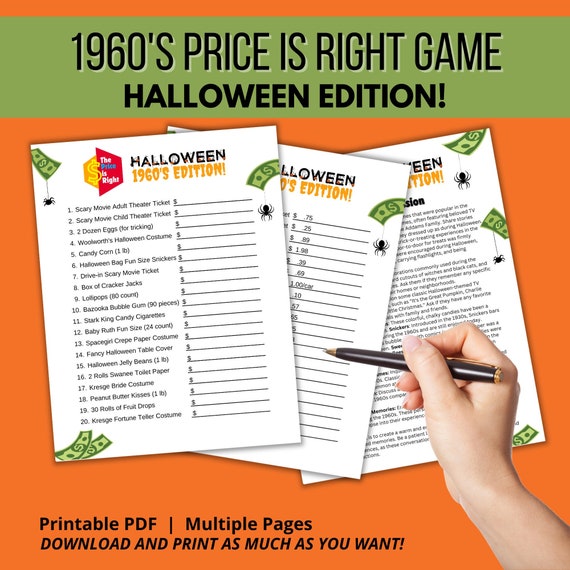The image is a vibrant promotional graphic for the "1960s Price is Right Game, Halloween Edition." The background is a striking orange, and a green banner at the top prominently displays the game title in bold, black lettering. Beneath this banner, three sheets of paper are artfully spread out and partially overlapping. The fully visible top sheet is adorned with a red box containing the text "The Price is Right," accompanied by a yellow dollar sign set against a small yellow background, emphasizing the Halloween-themed 1960s edition. This page outlines various questions or information pertinent to the game. Additionally, the sheet highlights, in black text, that the file is a printable PDF consisting of multiple pages, noting it can be downloaded and printed as often as desired. This carefully detailed depiction entices viewers to explore and engage with the nostalgic, festive game offering.